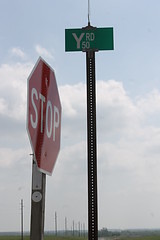In this vivid close-up image, the iconic red stop sign, featuring the bold white word "STOP" centered and outlined by a white trim along each corner of its octagonal shape, is prominently displayed. The sign is mounted on a sturdy silver metallic pole, likely stainless steel, ensuring visibility and durability. Positioned to the right of the stop sign, a taller silver pole with a green street sign at the top indicates "Y Rd 50" in white lettering. Above the street sign, there is a curious, thin post whose purpose is unclear. The sky behind the signs is a picturesque expanse of deep blue, dotted with numerous fluffy white clouds. In the background to the right, a series of telephone poles march into the distance, and the horizon is adorned with a touch of greenery from grass and distant trees.